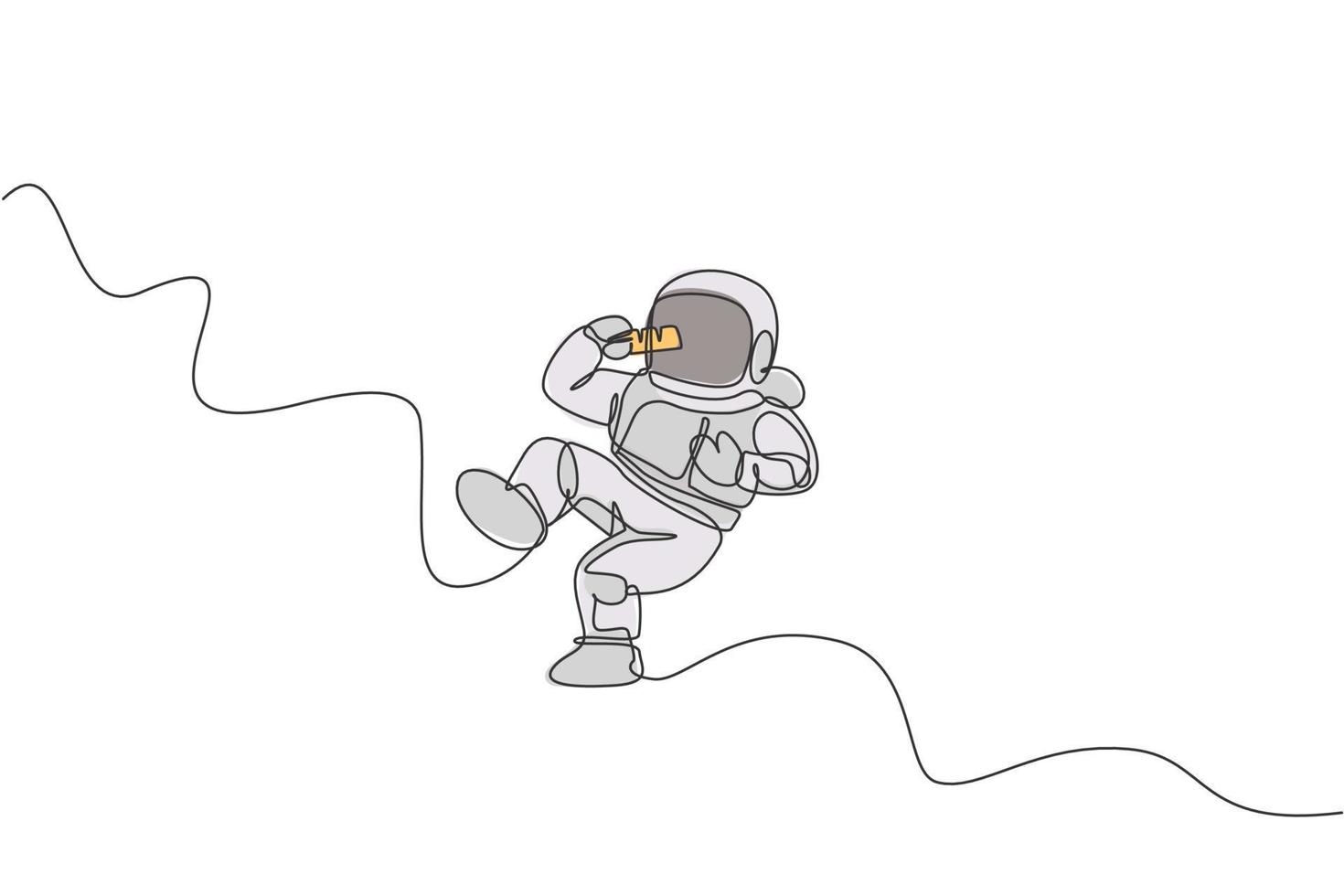A simplistic cartoon drawing depicts a spaceman on a stark white background. The astronaut, dressed in a gray and silver suit with a non-transparent helmet, appears to be clutching a pair of yellow sunglasses against the dark visor. His suit, although bulky around the torso with what seems like rolls of blubber at the back of the neck, contrasts with his disproportionately small legs. Notably, his left hand has just two fingers, while the right hand resembles a claw. The spaceman is interacting with a continuous black line starting from his right foot that threads up and down across the image, connecting to the top left corner and bottom right, suggesting he might be climbing or suspended in space. His posture is leaned backward, creating an illusion of either floating or falling in the void, adding a touch of dynamic tension to the otherwise minimalistic illustration.